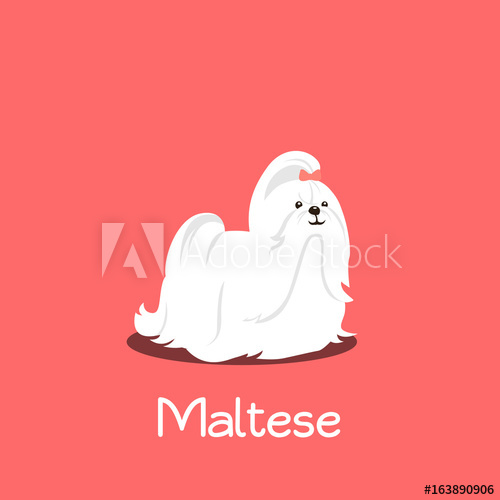This image features a white, shaggy Maltese dog centered against a peach-colored background. The dog's fur is long and drapes down to the ground, with a tuft of fur arching over its forehead. It has expressive black eyes, a black nose, and a slightly curled black mouth. Overlaying the image is a semi-transparent watermark that includes the Adobe logo and the words "Adobe Stock," indicating that this is a stock photo. Below the dog, in white font, is the caption "Maltese." Additionally, at the bottom right-hand corner, the image is marked with the number "163890906" in black font. The overall tones of the image are peach, white, and black.